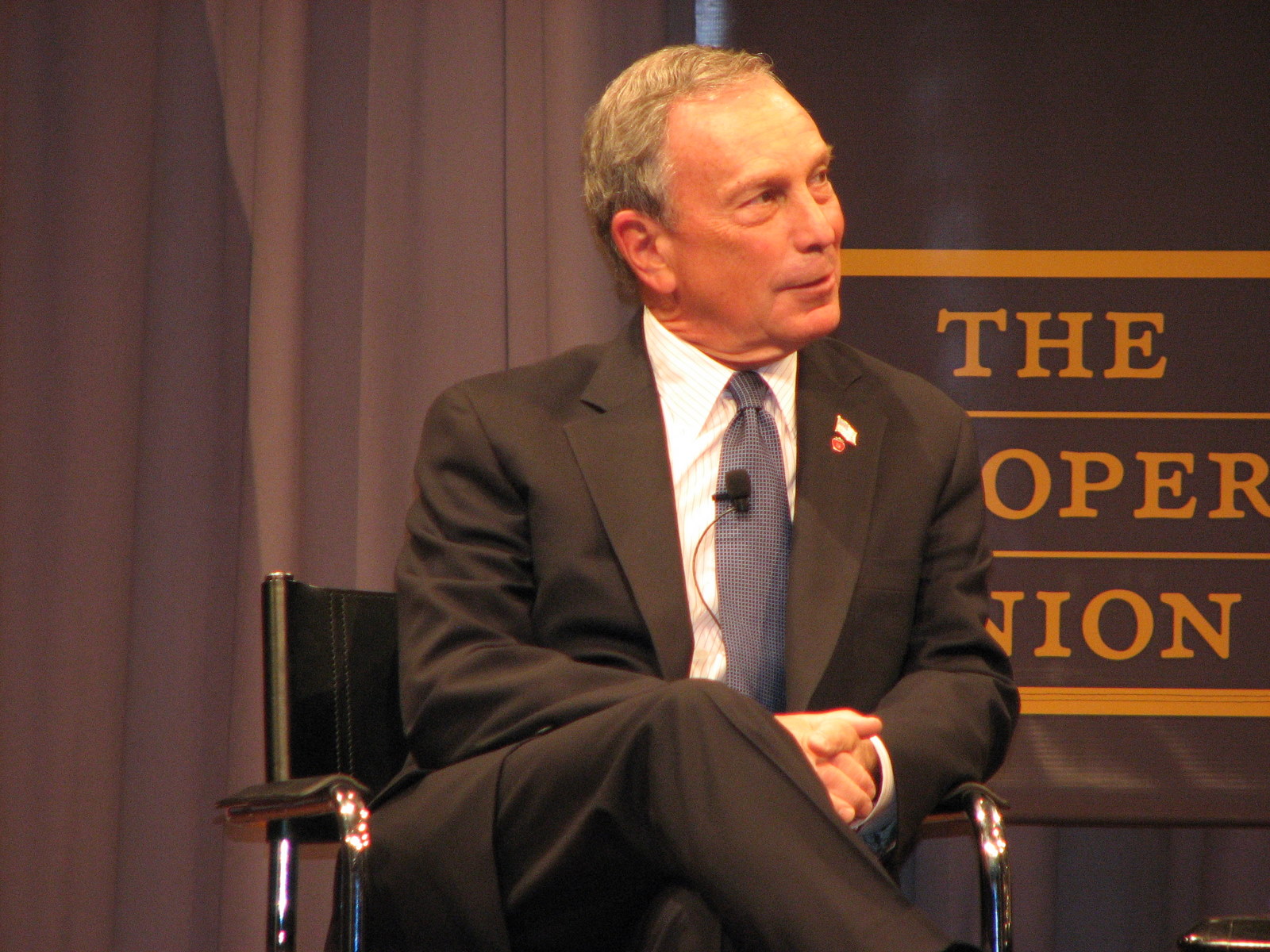In this detailed close-up image, an older gentleman with neatly combed, silver hair can be seen sitting in a black leather chair with metal armrests that have leather padding. He is dressed in a dark grey suit paired with a white collared shirt and a grey tie with a small check pattern. A microphone is clipped to his tie, and an American flag pin adorns his lapel along with a red pin beneath it. His legs are crossed as he looks slightly to his left, appearing to engage with someone perhaps on a higher plane, like in a talk show setting. The backdrop includes a prominent grey curtain over his right shoulder and a black banner with gold lines and partial text over his left shoulder, which reads "OPR" and "NION." The man has a pleasant expression with a slight smirk and noticeable bags under his eyes.